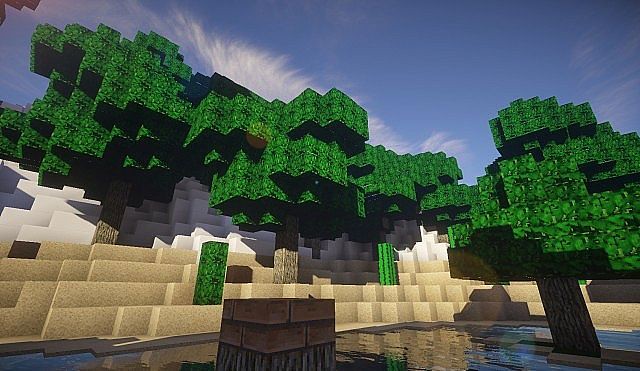This image is a screenshot from the game Minecraft. It features a clear body of water, displaying hues of blue and gray, possibly representing a lake or a pool. In the center of the image is a large, round structure lined with gray, round bricks stacked horizontally. Surrounding this structure, there are tan-colored blocks that step upwards, resembling a sandy beach. Dotting the landscape are trees made up of multi-colored green cubes, with rectangular brown trunks that have a bark-like texture. One tree even emerges from the water, which reflects the surrounding elements. The left and right sides of the image feature stacks of dark green rectangular boxes, resembling bushes or shrubs. In the background and above the trees, white and light gray blocks suggest buildings or clouds. The sky is a vibrant blue, adorned with wispy white clouds, evoking a serene and animated atmosphere.